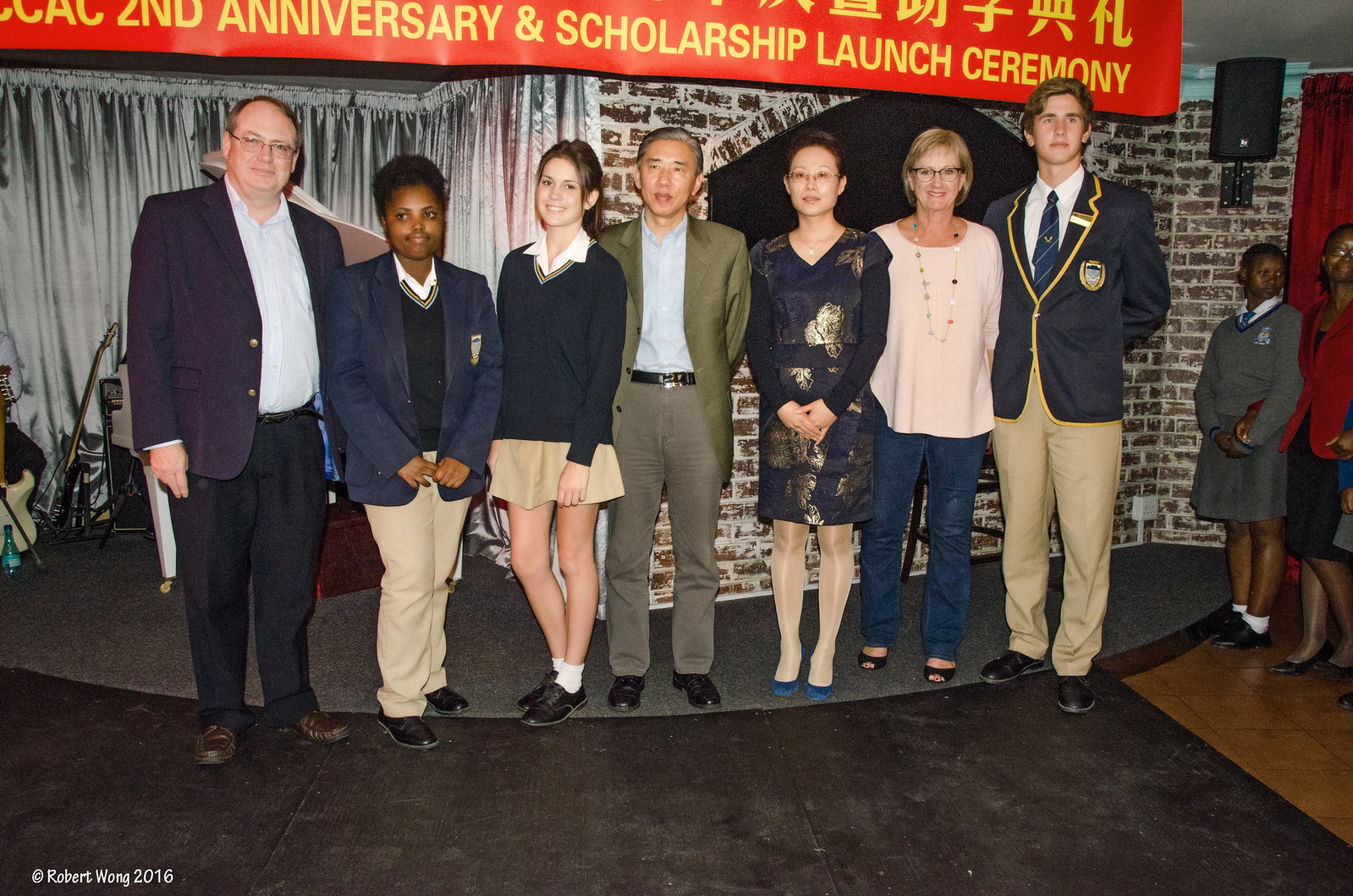The photograph shows seven people posing on a small stage, likely at some sort of event center. The backdrop features a big red banner with yellow text reading "CAC Second Anniversary and Scholarship Launch Ceremony," accompanied by Chinese characters above it and a silver curtain behind a faux brick wall. In the lower left, "Robert Wong 2016" indicates the year and perhaps the photographer or organizer.

The seven individuals stand in a mix of business casual attire that prominently features blue blazers and khaki tan clothing. On the left, there is a middle-aged man, the second tallest in the group, wearing a dark jacket, light-colored button-up shirt, grey slacks, and brown shoes. Next to him is a young black girl in a blue blazer with an emblem, a V-neck sweater with orange and green accents, khakis, and black tennis shoes. She is holding her fingers in front of her and looking to her right. 

To her right, another girl is wearing a short khaki skirt and a similar V-neck sweater. An Asian man and woman stand next to this young girl, while at the far end of the group is a middle-aged white woman and a very tall young man. This young man, seemingly college-aged, is wearing a blazer with the same insignia as the first girl, detailed with gold hems, khaki pants, a white button-down shirt, and a tie.

The scene suggests they might be participants or honorees at this scholarship launch ceremony, standing in front of a waiting line of others ready for their turn.